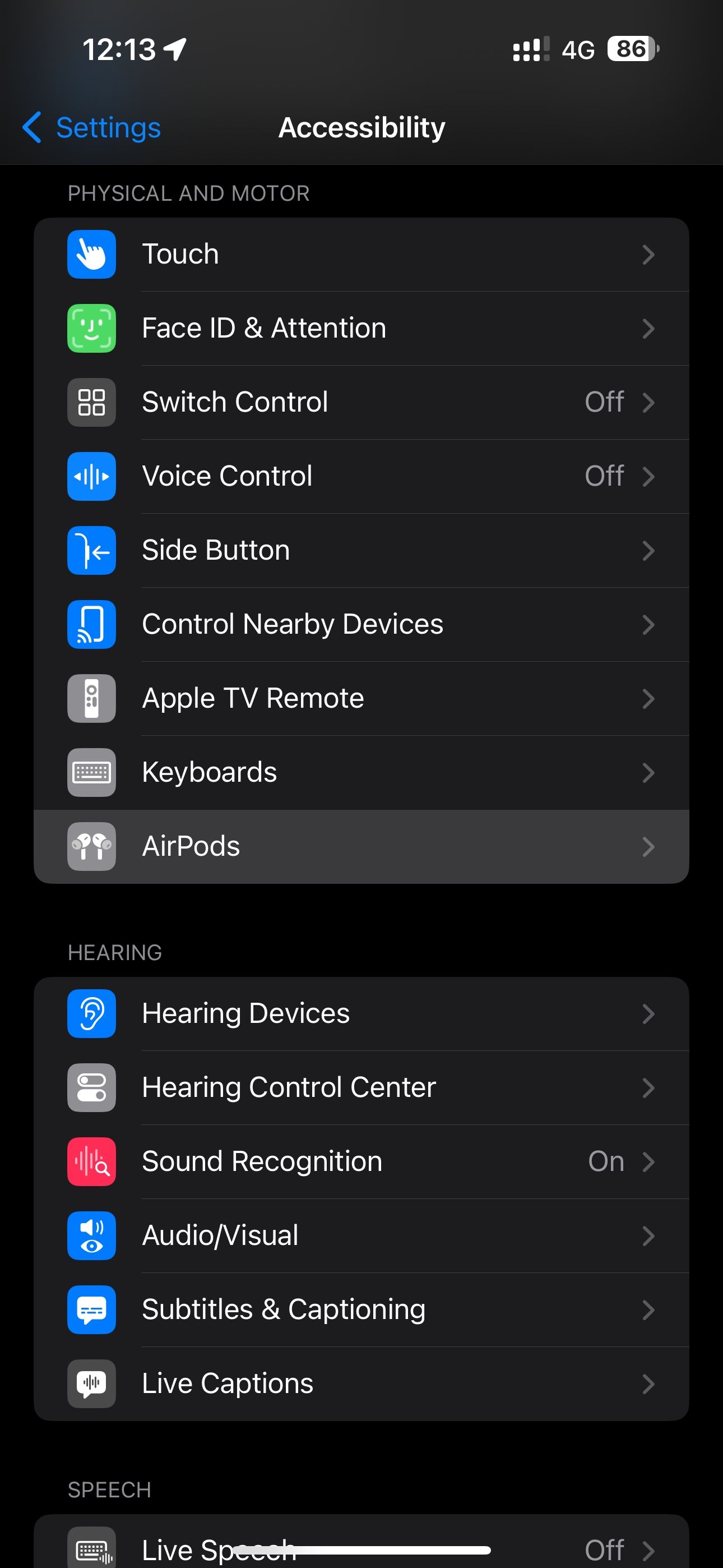The image features a dark background with various elements depicting a device accessibility settings screen. At the top, the status bar displays "12:13" in white, an arrow pointing to the upper right, several small dots, the "4G" signal strength, and "86" inside a white box.

Below the status bar, the title "Settings" is shown in blue with a leftward arrow. The word "Accessibility" is written in white underneath. Below this, the heading "Physical and Motor" appears in a faint font. The following items are listed:

1. **Touch**: Displayed in a blue box with a hand icon.
2. **Face ID & Attention**: Shown in a green box with a white face icon.
3. **Switch Control**: In a black box marked "off" with a small arrow beside it.
4. **Voice Control**: In blue with a white voice icon.
5. **Side Button**: Also in blue.
6. **Control Nearby Devices**: Displayed as a blue button with white inside.
7. **Apple TV Remote**: Shown in gray.
8. **Keyboards**: Gray with a keyboard icon.
9. **AirPods**: Gray with an AirPod icon.
10. **HEARING**: Listed category with sub-options below.

   - **Hearing Devices**: In a blue box.
   - **Hearing Control Center**: In a gray box.
   - **Sound Recognition**: In a red box, marked "on".
   - **Audio/Visual**: In a blue box.
   - **Subtitles and Captioning**: In a blue box.
   - **Live Captions**: In a black box with a white rectangle inside.
    
Lastly, the section titled "Speech" contains "Live Speech" marked as "off," with little arrows adjacent to each setting.